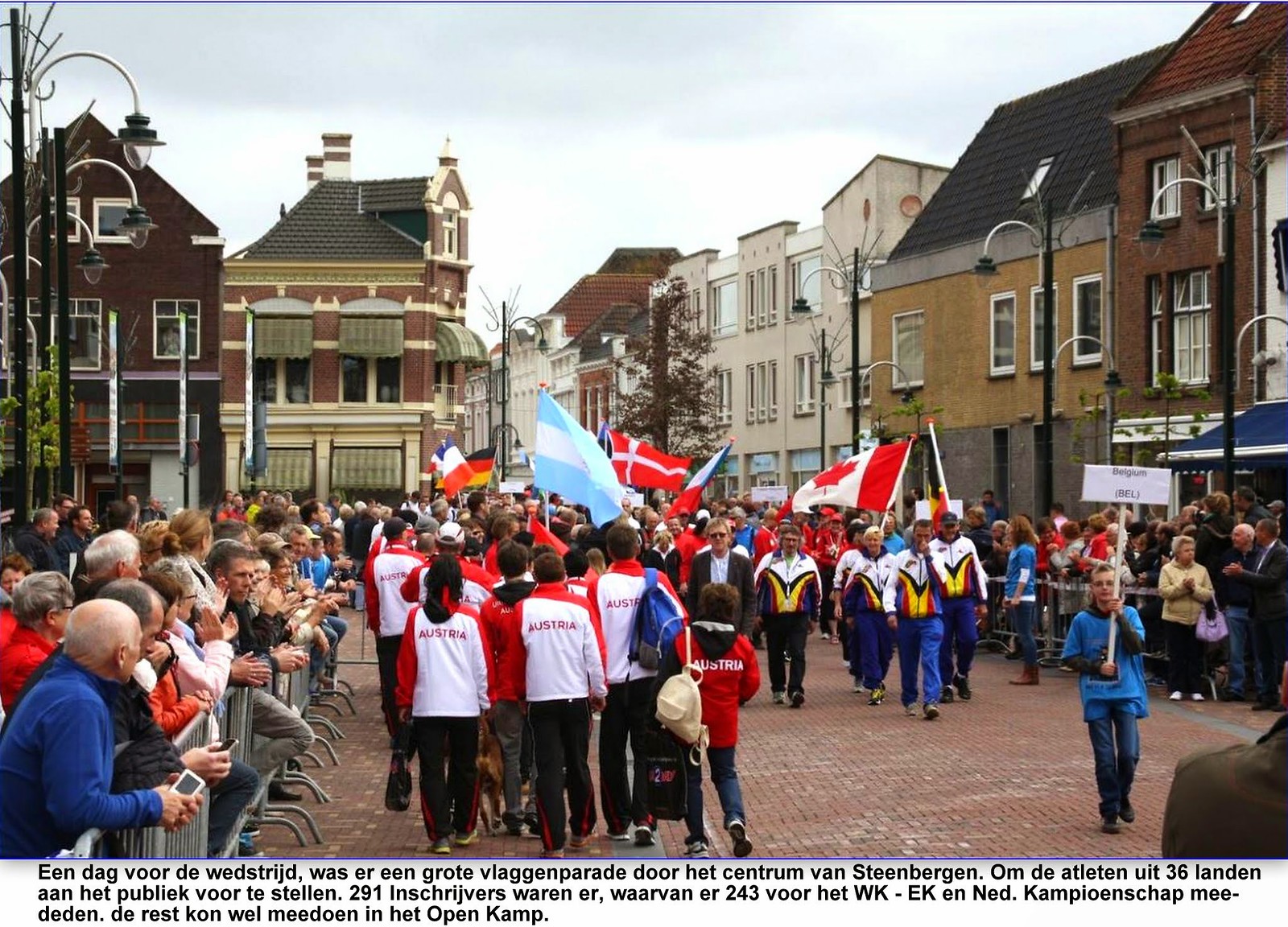The photograph, taken outdoors during the daytime, captures a vibrant parade-like event set along a beautifully preserved brick road flanked by older-style, three-story buildings tightly packed together, reminiscent of an old European town, possibly in Austria. On both sides of the road, metal barricades hold back crowds of people clapping and watching the proceedings with great interest. 

Two distinct groups are visible in the center of the street. The group on the left wears white shirts with long red sleeves, and "Austria" written on the back in red print. They are holding up Austrian flags proudly. On the right side, a sign carried by a child reads "Belgium (B-E-L)," leading a group dressed in yellow, blue, and white jumpsuits. Various other national flags, including those of Canada and Germany, add to the international atmosphere of the event.

Details in the photograph reveal an inscription in a foreign language at the bottom in black print, though its exact content remains unclear. The cloudy gray-blue sky serves as a backdrop to the picturesque, continuous row of tall, historic buildings lining the road, which could be either residential or commercial in nature. The lively and cheerful ambiance, along with the international representation, suggests a festive celebration bringing together diverse communities, possibly a sports event or cultural parade.